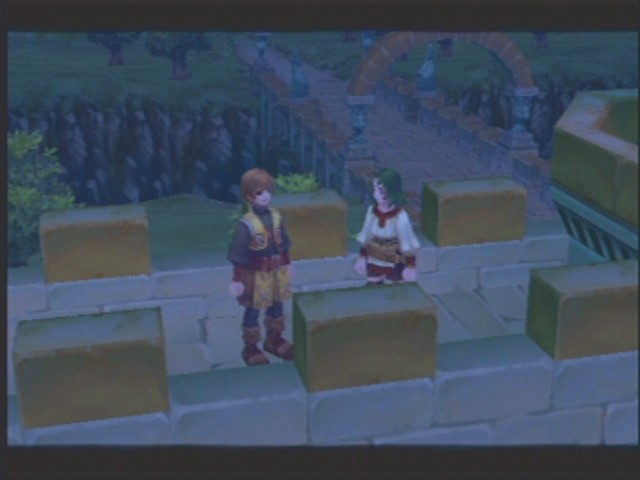This image is a photograph of a paused video game, resembling a scene from Legend of Zelda or a similar title. The focal point is two characters standing on a stone parapet that strongly resembles the Great Wall of China. The wall is constructed from alternating large gray and brown rectangular blocks, with brown blocks spaced intermittently like teeth along the edge. The left character, who has light skin and brownish-gold hair, wears traditional Chinese robes consisting of a gray top, darker bottoms, and a vest in shades of yellow and reddish-burgundy, complemented by matching footwear. The right character, donning greenish hair, is dressed in a light-colored top with a red collar, red and white bottoms, and similarly styled traditional attire. Both characters have ornate collars, wide belts, and poofy sleeves, underscoring their classic and youthful appearance. They face opposite directions, with one facing right and the other left, as they stand centrally on the stone walkway. The background on the left features rocks and a field, transitioning into a stone path with an archway that extends towards a distant forest on the right. The image appears to be a photograph of a computer monitor, as indicated by the visible black cell borders at the top and bottom edges.